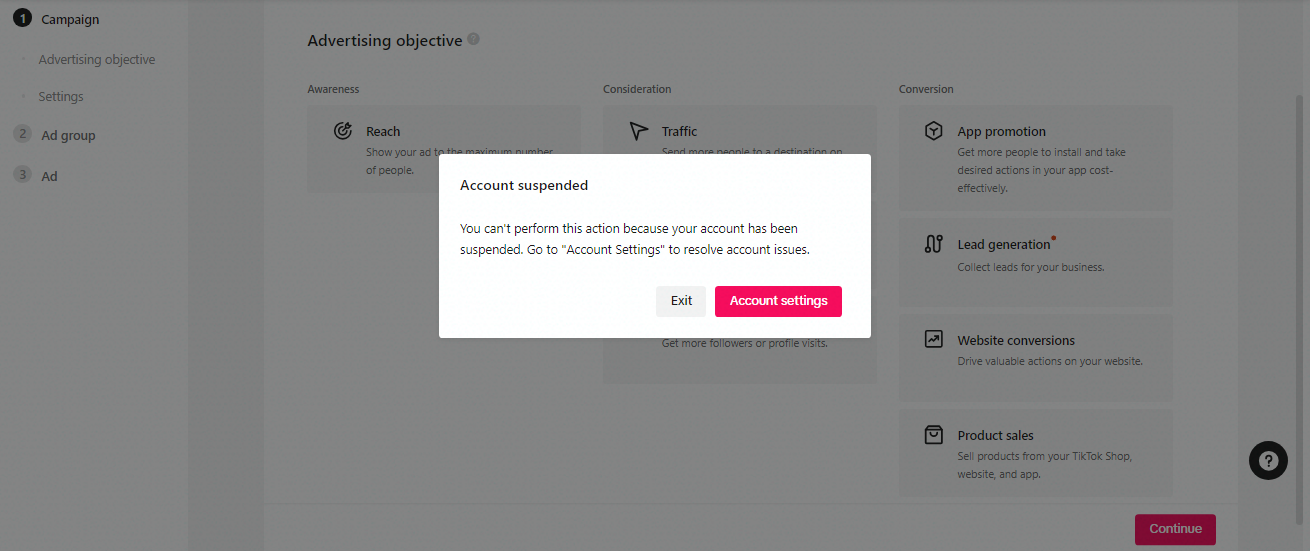A screenshot captures the back end of a webpage designed for advertising management. Dominating the screen is a prominent pop-up box that alerts the user with a message in black font against a white background. The message reads: "Account Suspended. You can't perform this action because your account has been suspended. Go to account settings to resolve account issues." Below this message are two buttons: one white button labeled "Exit," and a bold red button labeled "Account Settings."

Although the contents behind the pop-up are partially obscured, a few elements are still visible. The top left corner of the screen displays a navigation menu featuring options such as "Campaign," "Advertising Objective," "Settings," "Ad Group," and "Ad." In the center third of the webpage, the section titled "Advertising Objective" is partially observable, displaying icons and text for various objectives. These include "Reach" with a target icon, "Consideration" with a traffic icon, "App Promotion," "Lead Generation," "Website Conversions," and "Product Sales." However, the details are mostly muted due to the account suspension notification blocking the view.